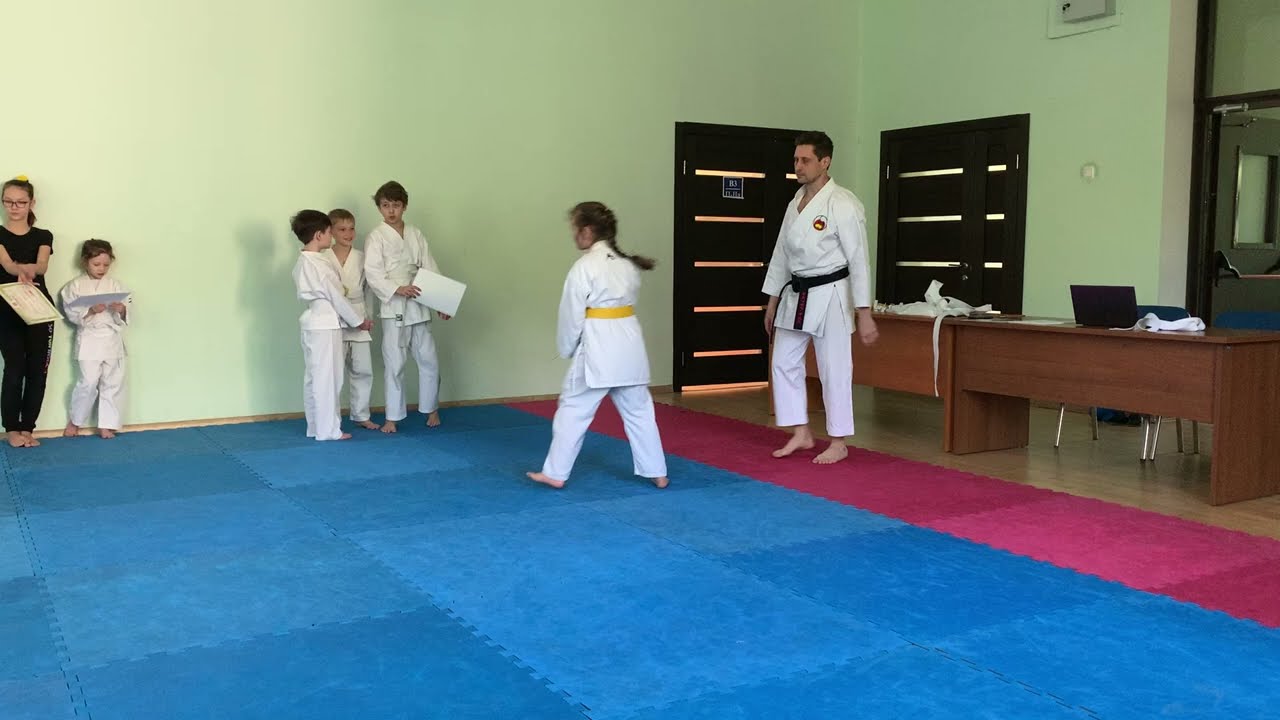In an indoor karate school with light green walls and a floor of interlocking blue and red foam tiles, a karate class is in session. At the center stands a young woman wearing a white karate gi with a yellow belt, looking off to the left. The instructor, a man with a black belt, also in a white gi, is positioned on the right side of the frame. Behind him, a long desk with a laptop is visible, alongside a corner with black panels and orange and white lighting.

Against the wall to the left of the young woman are four children, aged approximately 8 to 13, all barefoot and dressed in white karate outfits. One is an older boy in pure white, and another is a younger boy engrossed in something he's holding. To their left stands an older teenage girl or adult woman in dark clothing and glasses, holding what appears to be a bag or book. Everyone in the room, including the instructor and students, is barefoot. In the background, beyond the desk, are two doorways leading out of the room.